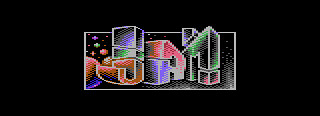The image is a piece of pixel art depicting the word "JAM" in 3D letters within a predominantly black, horizontal rectangle. The rectangle frames the image, which takes up roughly half of the total area. The background features a space-like theme with various colored spheres resembling planets. In the top left corner, there are circles in purple, green, red, and orange. The word "JAM" is spelled out in capital letters, with each letter composed of multiple colors. The "J" is segmented into an orange, green, and purple gradient from top to bottom. The "A" features a blend of purple on the top and red on the bottom. The "M" is divided into three sections: the top left in purple, the middle in green, and the bottom right in red. The letters extend out of the frame slightly, enhancing the 3D effect of the artwork. The entire piece has a retro, pixelated aesthetic, reminiscent of early digital art or vintage video game graphics.